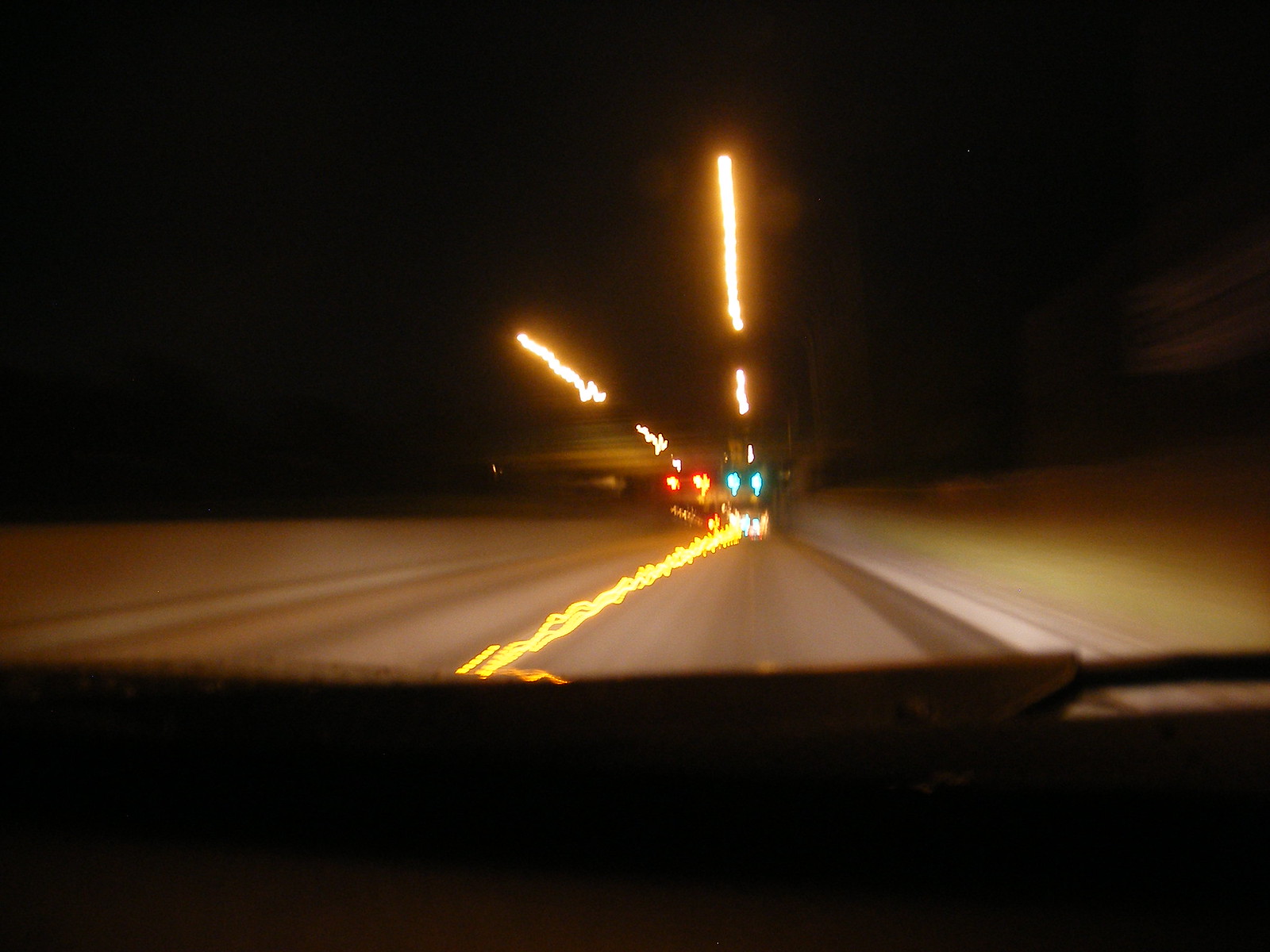This nighttime photograph, taken from inside a vehicle, likely from the passenger seat or via a dash cam, presents a captivating street view. The top of the image is dominated by a black sky, indicating the night setting. The lower quarter of the photo features a dark area resembling the vehicle’s dashboard. In front, the gray, slightly blurred asphalt roadway is marked by solid white stripes on both sides and a wavy bright yellow line down the middle. To the left, there is a gray divider, and on the right, a light slope with grass. The scene is dotted with various lights in the distance: white, green (probably traffic lights), and red (likely tail lights of vehicles ahead). Above the road, dashes of bright yellow lights, possibly streetlights, stretch into the sky, adding to the visual intrigue of the scene.